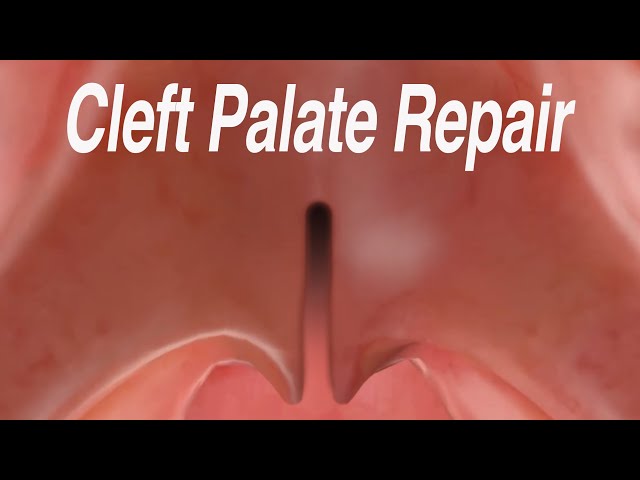The image, potentially used as a YouTube thumbnail for a "Cleft Palate Repair," features a distinct layout with black stripes on both the top and bottom. The central background is a deep reddish hue, overlaid with white text reading "Cleft Palate Repair." The background appears to be a computer-generated, highly zoomed-in depiction of the interior of a mouth, showcasing various shades of pink, red, and reddish-brown tissue. The image is somewhat out of focus, particularly in the upper left and right corners and in the depths, highlighting the complexity of the tissue textures. In the center, a vertical dark line runs through, suggesting the site of the cleft or perhaps a surgical repair. Despite the distorted and out-of-focus details, the image conveys its medical topic with emphasis on the mouth's interior environment.